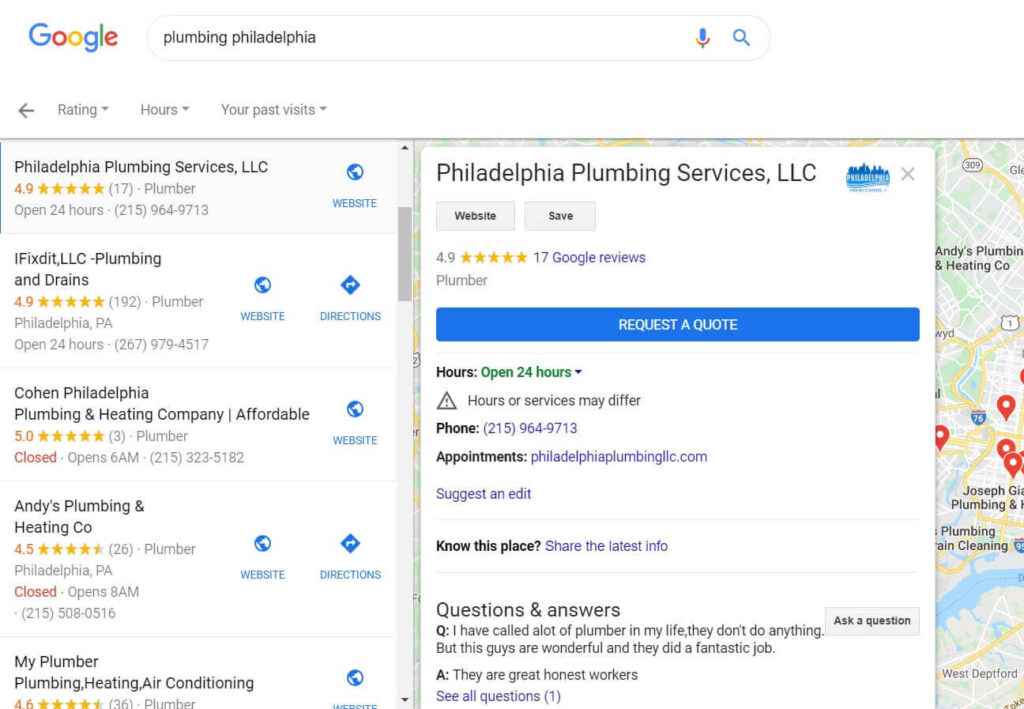This is a Google Maps screenshot displaying several companies relevant to the search query "Plum in Philadelphia." At the top of the screen, the search bar shows the entered query, followed by options to "Rate and review your past visit." Below, a dropdown menu with search results appears. The top search result is highlighted and expands into a detailed sidebar.

The sidebar provides an overview of "Philadelphia Plumbing Services LLC," featuring a website link, a save option, an impressive rating of 4.9 out of 5 stars based on 17 Google reviews, and a description label identifying it as a plumber. There is also a blue button labeled "Request a Quote."

Additional information includes the business's hours of operation, noted as "Open 24 hours," although it cautions that actual service hours may vary. The provided phone number for the business is 215-964-9713, with a link for booking appointments at PhiladelphiaPlumbingLLC.com. Users are encouraged to suggest edits. Below this, a message invites users to "Share the latest info," followed by a section for "Questions & Answers" with a button to "Ask a Question."